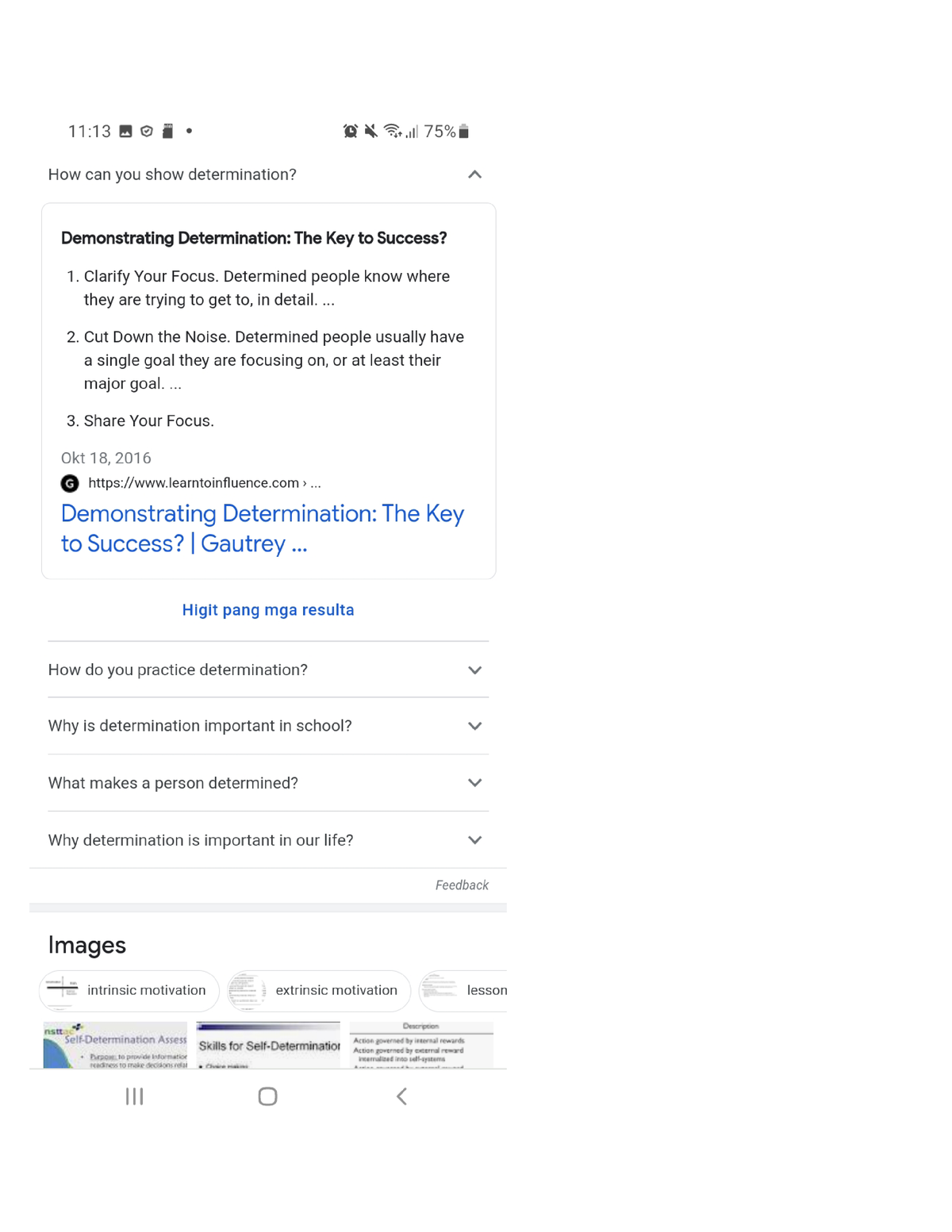A screenshot of a smartphone displaying an Instagram post is set against a white background with black text. At the top of the screen, the time reads 11:13. To the right of the Instagram logo, a series of icons indicate a shield, a SIM card, a dot, an alarm (sounds off), full Wi-Fi signal, near-full cellular signal, and a battery at 75%.

Centered on the screen in bold black text is the question: "How can you show determination?" Next to this, on the right, is an upward arrow. The text elaborates on this topic, describing three points as keys to success:

1. Clarify your focus. Determined people know exactly where they are aiming and detail their goals.
2. Cut down on the noise. These individuals concentrate solely on their main goals, avoiding distractions.
3. Share your focus.

Below this text is a timestamp in gray: "17, 2016." Accompanied by blue text, it reads "Demonstrate determination: the key to success," followed by a sentence in an unrecognized language.

Additional questions related to determination are listed:
- "How do you practice determination?"
- "Why is determination important in school?"
- "What makes a person determined?"
- "Why is determination important in our lives?"

Further down the screen are thumbnails of various images, though the details are largely obscured due to their small size.

At the bottom, three icons appear in gray: three horizontal lines, a square in the center, and a leftward-pointing arrow, suggesting navigation options.